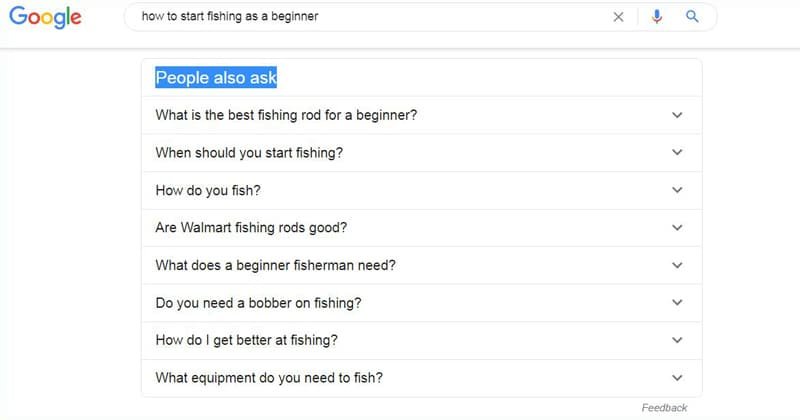The image is a screen capture of a Google search page. At the top of the image, the iconic Google logo is prominently displayed, featuring a blue "G", a red "O", a yellow "O", a blue "G", a green "L", and a red "E". Below the logo, a white search box is visible, containing the text "how to start fishing as a beginner" in gray, accompanied by a gray 'X' on the right side and a gold, red, and blue microphone icon on the left. Adjacent to the search bar is a blue magnifying glass icon.

As we move down the image, there's a section highlighted in blue with the text "People also ask" in white font. This section presents a series of related questions, each separated by thin gray lines and featuring a drop-down arrow for further expansion. The questions listed are:
1. What is the best fishing rod for a beginner?
2. When should you start fishing?
3. How do you fish?
4. Are Walmart fishing rods good?
5. What does a beginner fisherman need?
6. Do you need a bobber on fishing?
7. How do I get better at fishing?
8. What equipment do you need to fish?

At the very bottom of the visible section, there is the word "Feedback" in capital letters.

The overall image quality is decent, though there is slight pixelation, particularly noticeable around the microphone icon at the top. Despite this, the black font used for the search results is clear and easy to read. The image predominantly features text, with no significant visual distractions aside from the slight pixelation.